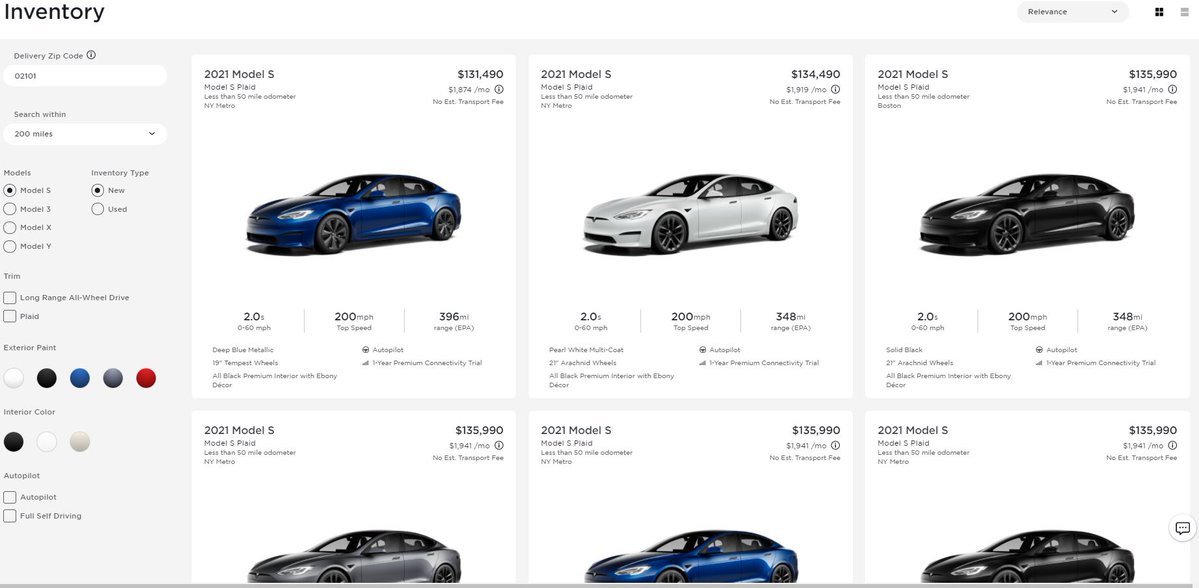**Detailed Caption for Car Company Website Screenshot:**

The screenshot captures the user interface of a car company's inventory browsing page, showcasing a detailed search and filter system specifically for Tesla vehicles. On the left sidebar, users can refine their search by entering a delivery zip code and setting a search radius, which in this case is configured to 200 miles. 

Below the search radius, users are presented with options to filter by model and inventory type, with choices including "New" or "Used" and available Tesla models: Model S, Model 3, Model X, and Model Y. Subsequent filters allow for selection of vehicle trims, with options visible as “Long Range All-Wheel Drive” or "Plaid" (albeit in small text).

Further customization is possible through the "Exterior Paint" section, offering color choices represented by five small circles in white, black, blue, gray, and red. The “Interior Color” section follows, providing three color options: black, white, or beige. Under the "Autopilot" section, users can choose between "Autopilot" or "Full Self-Driving."

In the main viewing area, the grid of car listings is prominently displayed. Each car tile includes an image of the vehicle, its model year, color, price, and key statistics. For instance, the first car listed is a blue 2021 Model S priced at $131,490, followed by a white 2021 Model S at the same price, and a black 2021 Model S priced at $135,990. Each car listing is detailed with specific attributes to aid the buyer’s decision-making process.